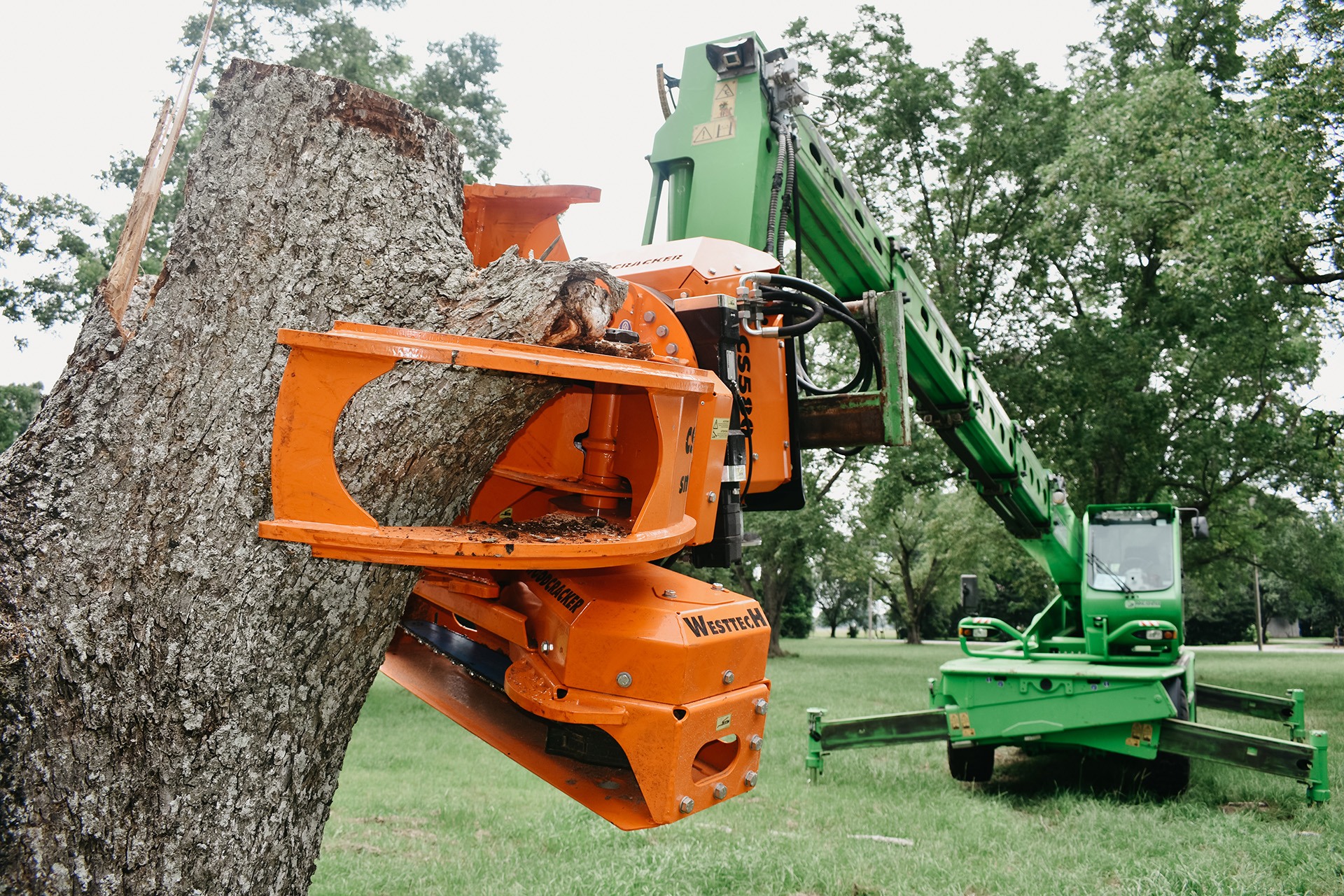The rectangular image captures an outdoor scene featuring a tree-trimming operation. Dominating the photograph is a green work vehicle equipped with a long arm and a bright orange gripping mechanism, likely a vice or clamp, which is firmly holding a partially lopped-off tree trunk. The vehicle, designed for precise tree maintenance tasks, includes a cab for the operator and a spotlight for nighttime or dim-area operations. The background features a park-like setting with a lush green lawn, multiple other trees with abundant green leaves, and a light, almost grayish-blue sky. This picturesque day shows the equipment diligently working amidst a spacious green field.